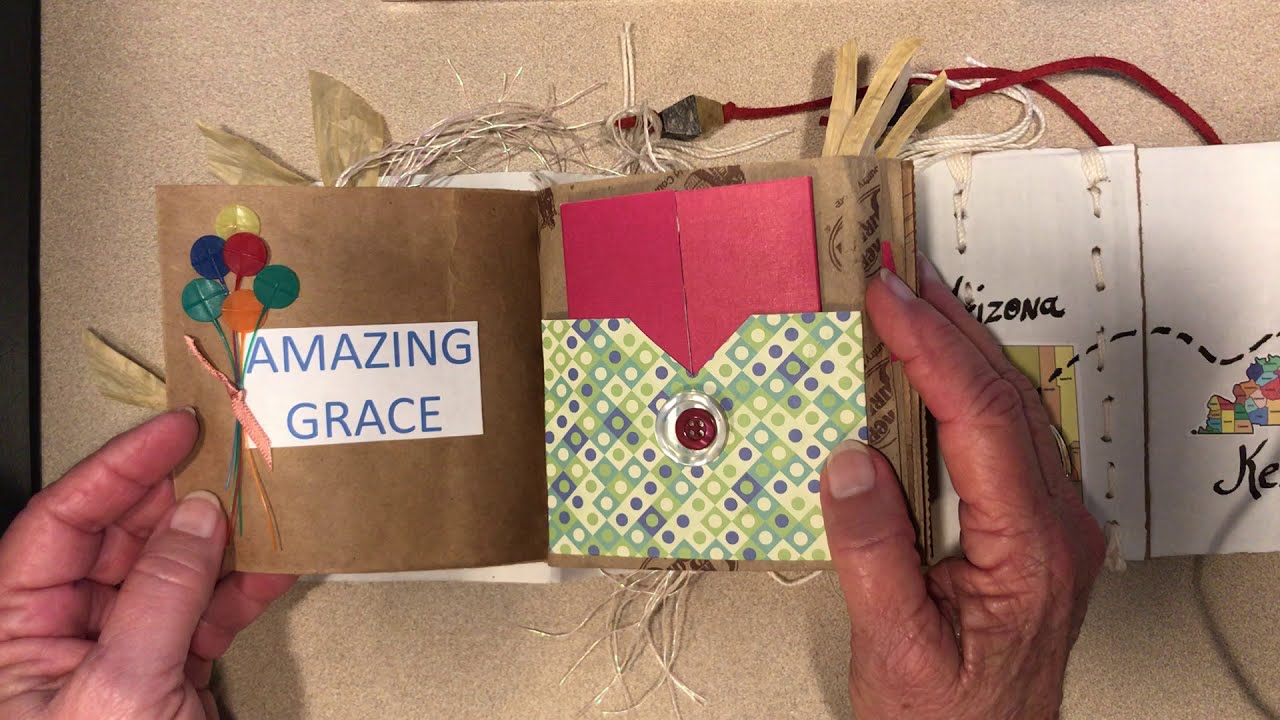The image depicts a pair of wrinkled hands holding open a small, handcrafted booklet indoors. The left page of the booklet features a white background with blue letters spelling out "Amazing Grace," adorned with whimsical orange, blue, and red balloon drawings tied with a pink ribbon. The background behind this page is a brown crepe-like paper. The right page contains a decorative green pocket with multicolored circular patterns, holding a red envelope. A red string extends horizontally across the top of the image, joined by a thin white string on the left. To the right of the person’s hands, additional booklets are pinned on what appears to be a corkboard, and a second open booklet reveals partial letters "I-Z-O-N-A" and "K-E," suggesting the word "Arizona." The scene sits on a speckled light brown surface, with a red cord and straw piece visible in the background, adding to the crafts-like atmosphere.